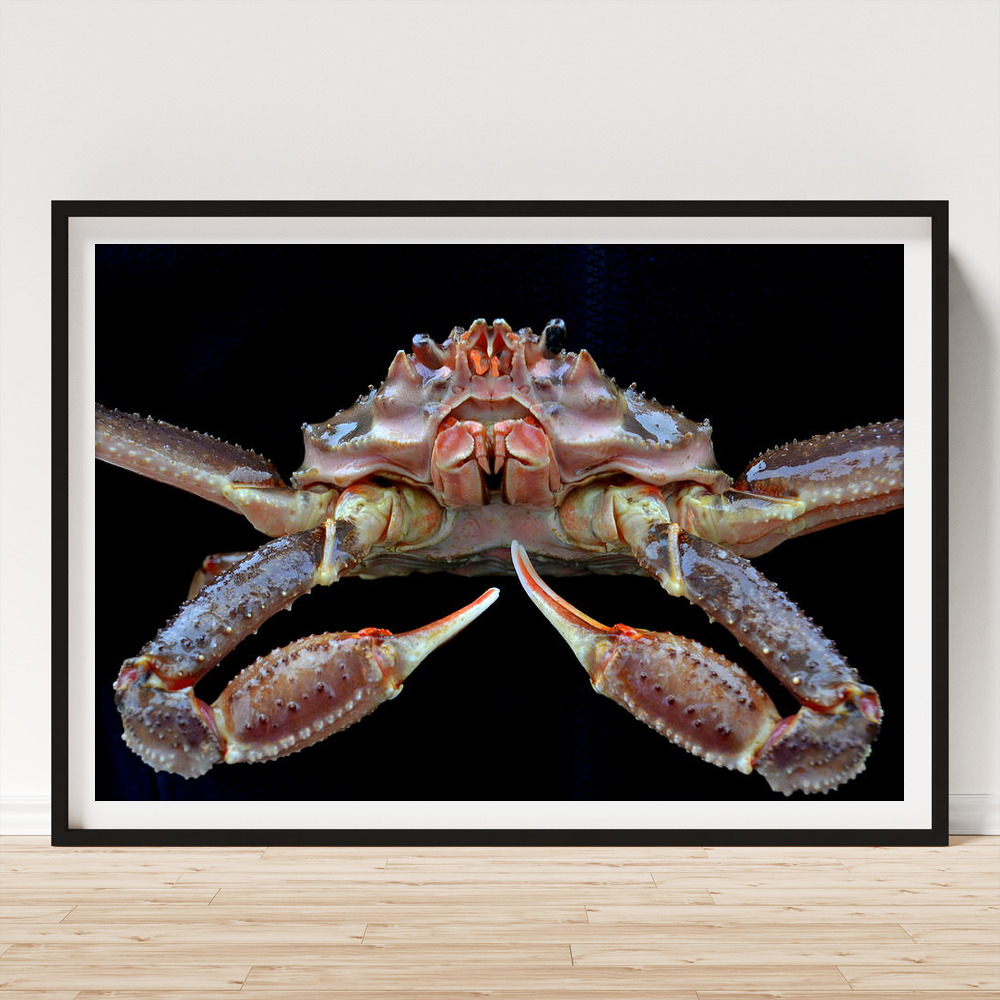The image showcases a framed artistic rendering or photograph of a crab, leaning against a cream-colored wall with a visible light beige wooden floor. The frame itself is thin, black, and likely made of wood, enclosing a white border. Inside the frame, a close-up of a crab is depicted against a completely black background. The crab features a realistic and detailed appearance, with visible pincers, partial legs, mandibles, eye stalks, and other anatomical features. The image's focus on the crab's face and front anatomy highlights its intricate details and vibrant colors, which include light purple, some pink, and blue hues. The overall setting gives the impression of a minimalist mock-up designed to feature the framed crab artwork prominently.